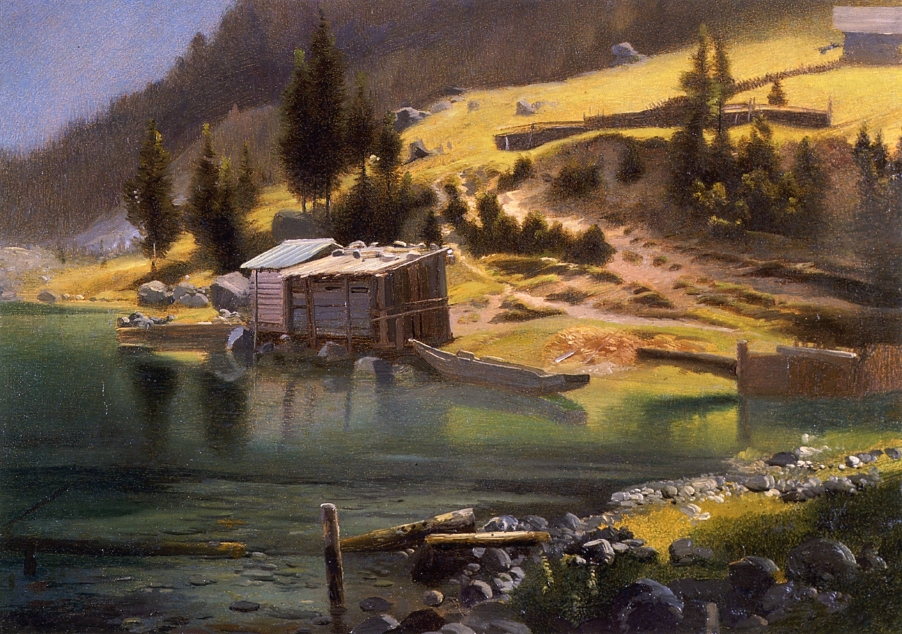This detailed painting, likely an oil work, captures a serene lakeside scene featuring a green-tinged lake lapping against a rocky shore. In the foreground, the water is clear enough to reveal submerged rocks and scattered, partially submerged wooden posts. On the grassy hillside bordering the lake, there is a small, rustic wooden shed right at the water's edge, flanked by two wooden boats, one a rowboat and the other resembling a canoe. The grassy hill, dotted with boulders, rises up to a fenced-in area partway up, leading towards another structure, possibly a barn, illuminated by sunlight. Surrounding this scene, a diverse forest of greens and browns encroaches upon the hill and lake, with some trees extending to the shed. The blue sky above holds a few white clouds, contributing to the tranquil atmosphere. The overall setting includes a mixture of grassy fields, rolling hills, and a distant tree line, suggesting a well-established, yet rustic lakeside area.